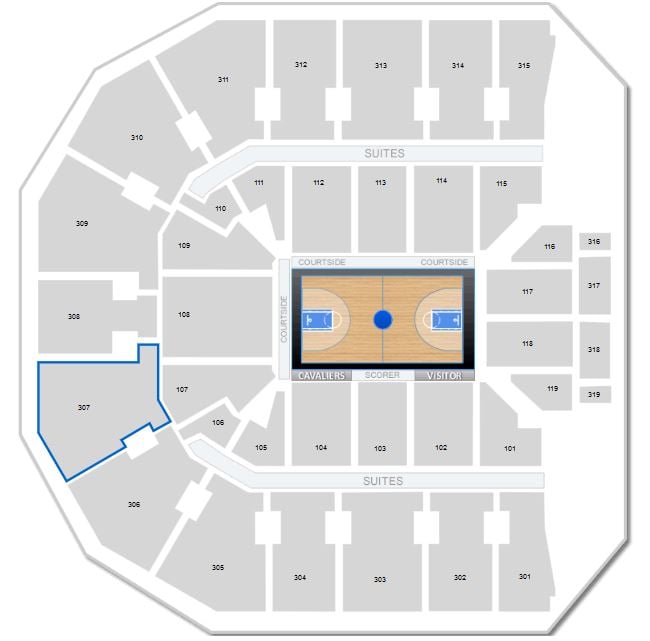This image showcases a detailed blueprint of a basketball gym layout, bordered by a gray outline that intricately traces around the gym's perimeter. The border begins approximately one inch from the top right edge, angling upwards towards the left and extending horizontally about three inches. It then descends downwards and leftward an inch before continuing in a downward slope to the edge, dropping around two inches. The border proceeds downward again about an inch, then again downwards to the bottom, continuing three inches horizontally across. It then moves up an inch to the right and ascends along the right side. 

Inside this gray border are numerous smaller sections. Starting from the right and moving left, there are five sections across the top, curving downward. One section is positioned upward left, with three sections descending along the left side. Another section is located to the left, with five sections spanning across the bottom. In the front rows of the top and bottom sections, there is a thin blue band labeled "Sweets." 

In the top section, there are five segments running across, two in the left corner, three descending along the left side, two in the bottom left corner, and four spanning across. The right side accommodates four segments, with an additional four segments situated closer to the right edge.

At the center of this layout is the outline of the basketball court, clearly marked with "Court Side" at the top and left side. The bottom is labeled with "Cavaliers," alongside the designations "Score" and "Visitor." Highlighted with a blue border, Section 307 is situated on the left side, specifically as the bottom section before reaching the left corner.